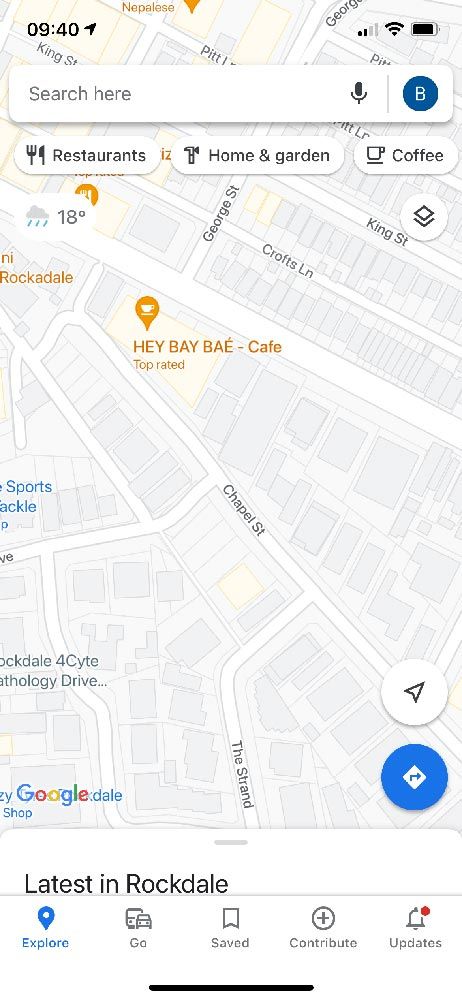This detailed description captures the essence of the image effectively. Here is a cleaned-up, detailed caption:

---

"A screenshot of a Google Maps interface on a smartphone. The top of the phone screen displays the time as 9:40 with a right-pointing arrow, indicating the strength of the Wi-Fi connection and full battery status. Below that, a search bar prompts 'Search here,' followed by various tabs labelled 'Restaurants,' 'Home and Garden,' and 'Coffee.'

In the central view of the map, a prominently marked, top-rated café named 'Hey Bae Bae Café' appears in gold. Surrounding street names include Chapel Street running diagonally, George Street running horizontally above Crofts Lane, which also runs horizontally, and King Street positioned at the bottom of the map section.

At the very bottom of the screen, Google's logo is displayed alongside several menu buttons: 'Explore,' 'Go,' 'Save,' 'Contribute,' and 'Updates,' each accompanied by its respective icon."

---